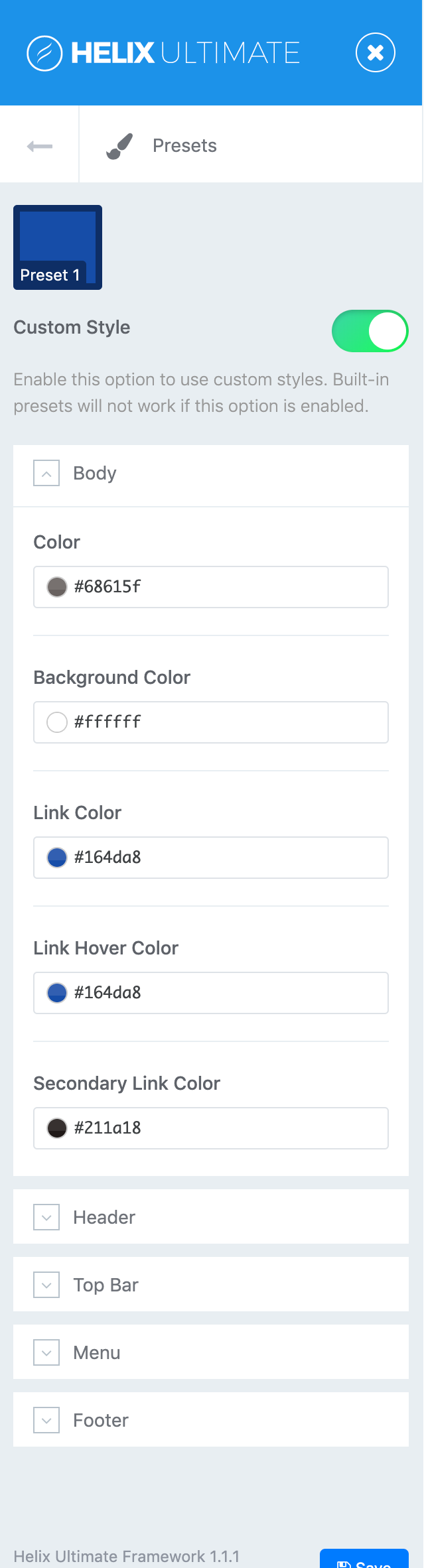This image capture portrays a settings page from a mobile device, displaying customization options for a template named "Helix Ultimate." At the top of the screen, enclosed in a blue rectangular banner, is the text "Helix Ultimate" in white font. Below this, the section labeled "Preset" lists different preset options, starting with "Preset 1," followed by "Custom Style" in gray font. The accompanying note informs users that enabling the custom style will disable built-in presets.

Beneath this, a green slider to activate custom styles is shown, with the slider positioned to the right, indicating that the feature is enabled. Further down, there's a “Body” category where users can specify a color. The entry for this field is "68615F,” and the background color is set to the hexadecimal value "#FFFFFF." Additional color customization options follow, including link color, link hover color, and secondary link color, among others, which can be individually set by the user.